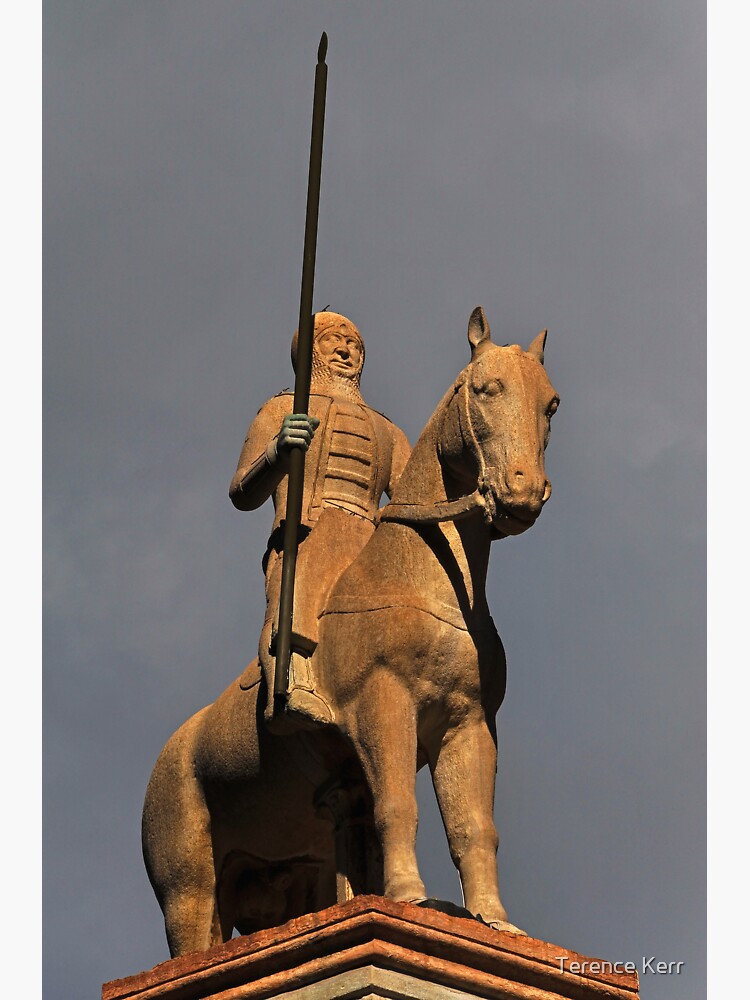The photograph captures a majestic statue by Terence Kerr, K-E-R-R, clearly marked at the bottom right. The image, taken from a low angle, emphasizes the grandeur of a warrior mounted on a horse, both rendered in a light brown, almost bronze-colored stone. The base of the statue is a square, brown pedestal, elevating the horse and its rider against a stormy gray sky. The warrior, clad in detailed armor with a chainmail headpiece, grips a long, spear-like object in his right hand, pointing it skyward. The horse, adorned with a bridle and chest harness, stands stoically with its head turned slightly to the right. Shadows, hinting at an external light source from the top left, create dramatic contrasts, particularly beneath the horse and around its neck. The overall composition and intricacy of the statue evoke a sense of medieval or possibly Asian-inspired artistry, combining historical reverence with artistic finesse.